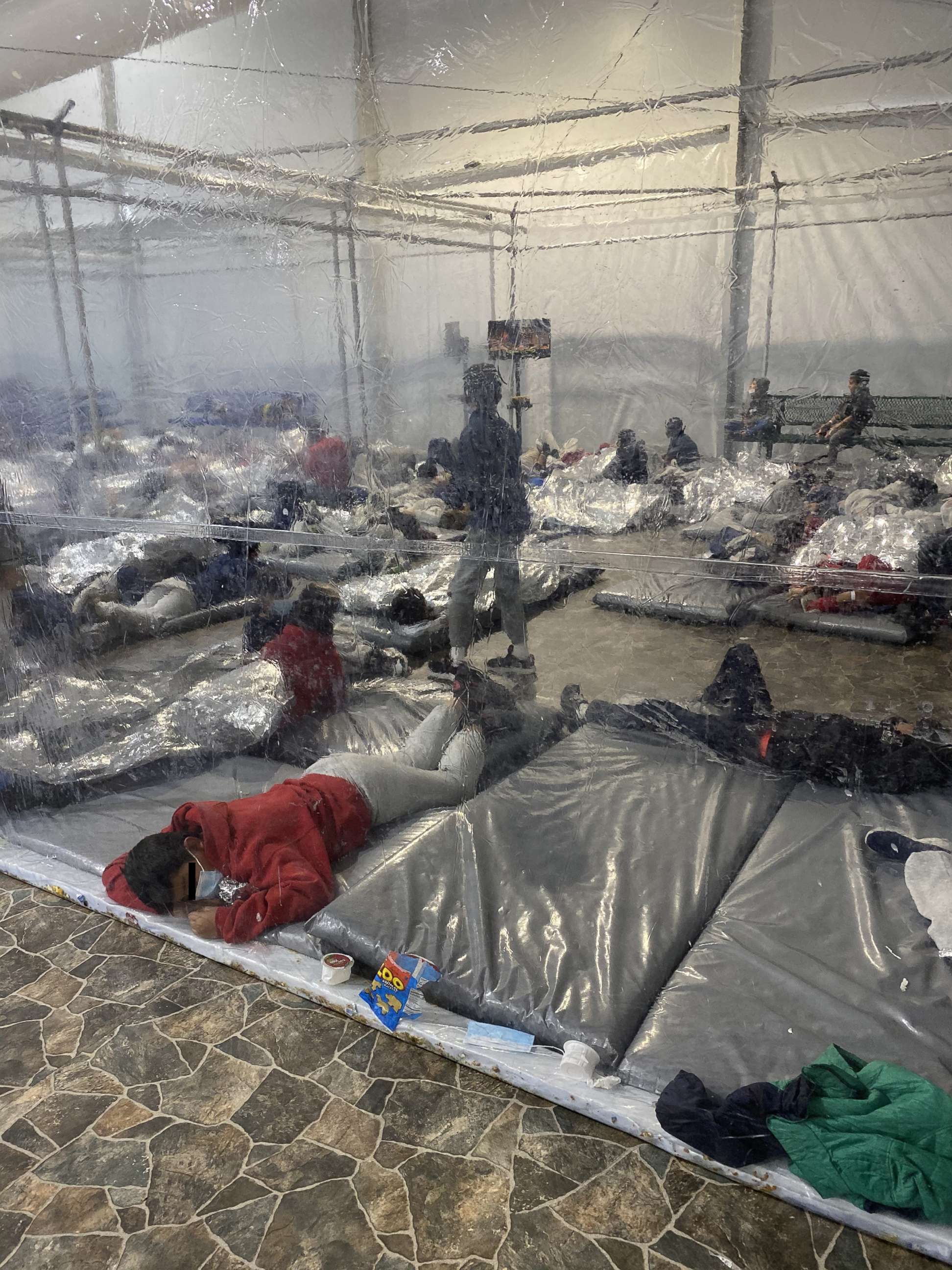This portrait-style photograph captures the interior of a detention center viewed through a glass panel. The scene is marked by rows of gray mats lined up on the stone-patterned floor, with several individuals laying on them, some wrapped in mylar blankets. A significant detail includes face masks scattered on the floor, and notably, a man in the foreground resting on one of the mats while wearing a face mask. Towards the back of the room, a bench seats what appear to be two children. A partially obscured sign is visible in the corner of the room, though its message is indiscernible. The overall atmosphere is somber and densely populated, highlighting the human aspect within the sterile environment of the center.